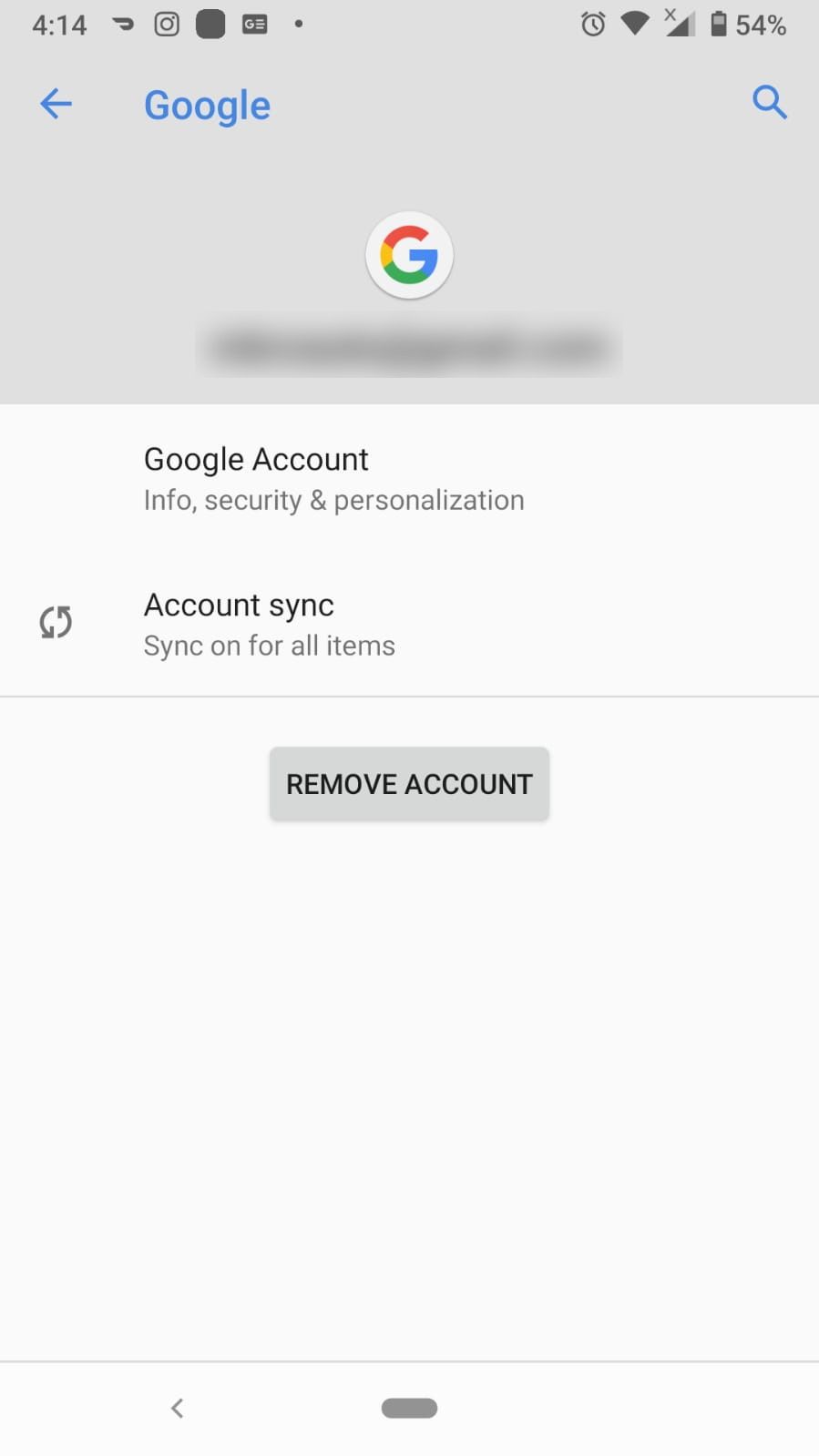**Detailed Caption:**

The image is a detailed screenshot of a Google Account page displayed on a mobile device. In the top-right corner, the battery icon indicates a 54% charge remaining. Adjacent to the battery icon, the cell service icon shows an 'X' above four bars, suggesting that the device is either not currently connected to a cellular network or that service is unavailable. To the left of the battery icon, there is a Wi-Fi symbol, indicating a strong internet connection. Further to the left, an alarm clock icon hints that an alarm is set on this device. The time displayed is 4:14.

On the home screen, various app icons are visible: the DoorDash icon, the Instagram icon, and a solid rounded-edge square icon. Additionally, there's a rectangular icon with a 'G,' likely representing Google News.

The main section of the page features a header with the Google logo, a back arrow on the left, and a search icon on the right. Below the Google logo, there is a blurred-out area obscuring the user's Google email address. The main title reads "Google Account," followed by three prominent sections: "Info, security and personalization," "Account sync," which shows that synchronization is enabled for all items, and a gray button labeled "Remove account."

At the bottom of the screen, there is a rounded gray oval and a visible back button, typical of a mobile interface, although the specific device brand or model is not discernible from this screenshot. The image clearly captures the user interface for managing a Google account on a mobile device, encapsulating various functionalities and settings available to the user.